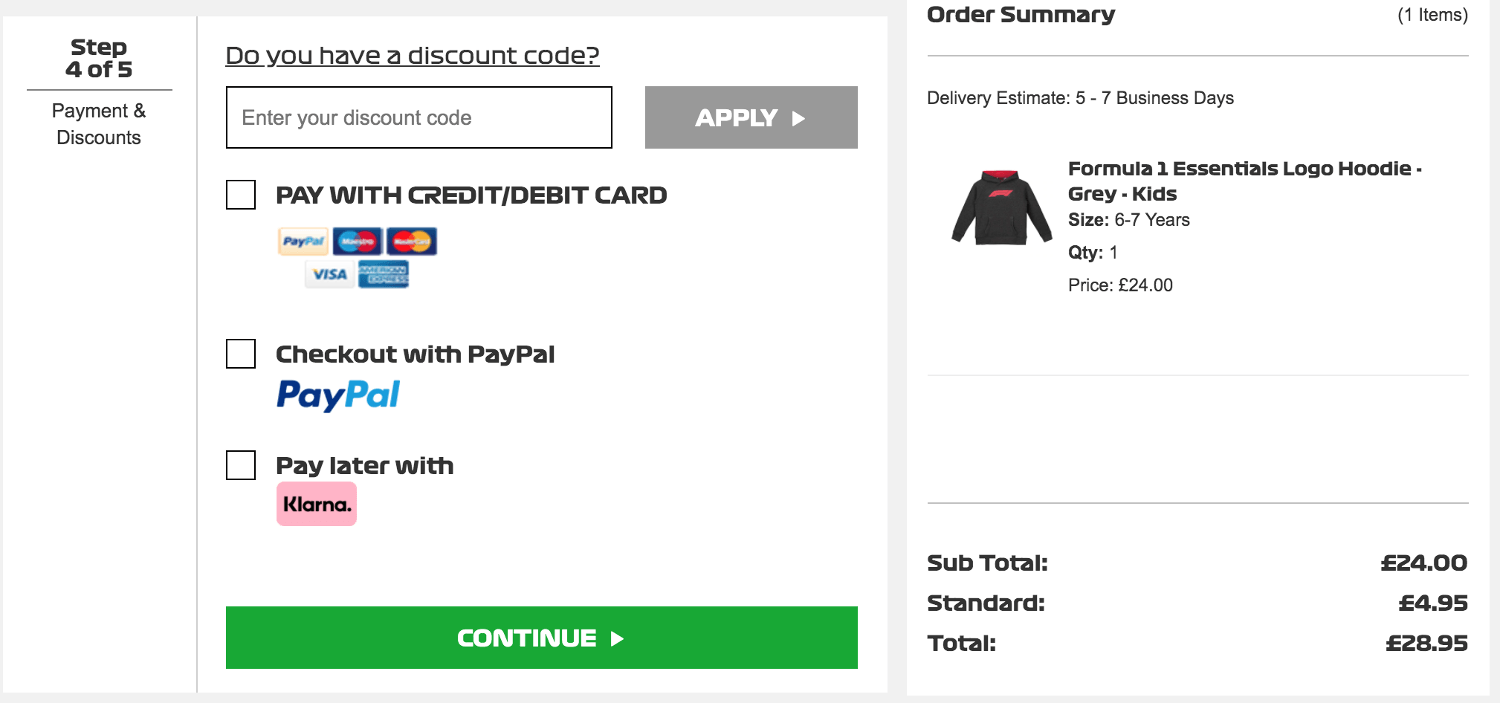A detailed checkout page screenshot is depicted, showcasing the final stages of an online purchase process. At the top left, it signifies "Step 4 of 5" in black font with a gray underline. Adjacent to this, the heading reads "Payments and Discounts," accompanied by an option to enter a discount code. 

Prominently displayed on the right is the prompt, "Do you have a discount code?" underscored for emphasis. Below this, there is a text box labeled "Enter your discount code," followed by an adjacent 'Apply' button.

The page features three neatly boxed payment options. The first box allows for payments via credit or debit cards, displaying icons for PayPal, MasterCard, American Express, and Visa. The second box offers a direct checkout with PayPal, marked by another PayPal icon. The third option, highlighted with a black "Klarna" label on a pink background, offers a "Pay Later with Klarna" service.

At the bottom, a green "Continue" button invites further progression in the checkout process. Notably, on the middle right side of the image, a product picture is visible, illustrating a gray hoodie with the "Formula One Essentials" logo.